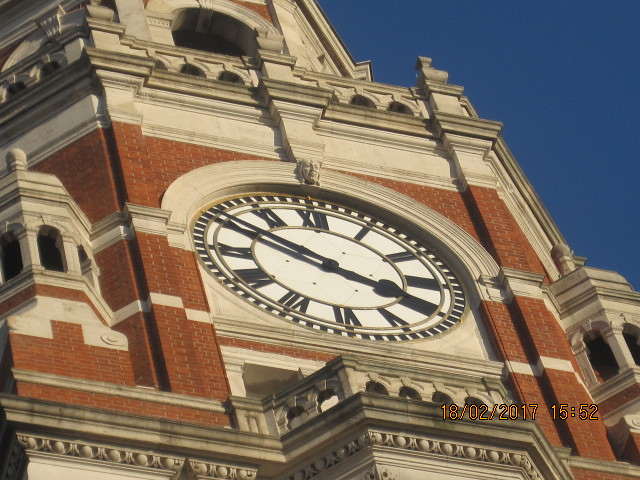This photograph captures an ornate, old-fashioned building facade prominently featuring a large clock embedded in its center. The clock face, which boasts a classic design with black Roman numerals and hands set against a stark white backdrop, commands attention. Above the clock, there is an intricately carved stone face, adding to the building's historical charm. The structure, constructed from bright orange bricks and accented with light tan and gray stone details, stands out brilliantly against the dark blue sky. In the bottom right corner of the image, retro orange text displays the date and time as "18-02-2017 15:52". This meticulously detailed clock and the richly decorated architectural elements evoke a sense of timeless elegance and grandeur.